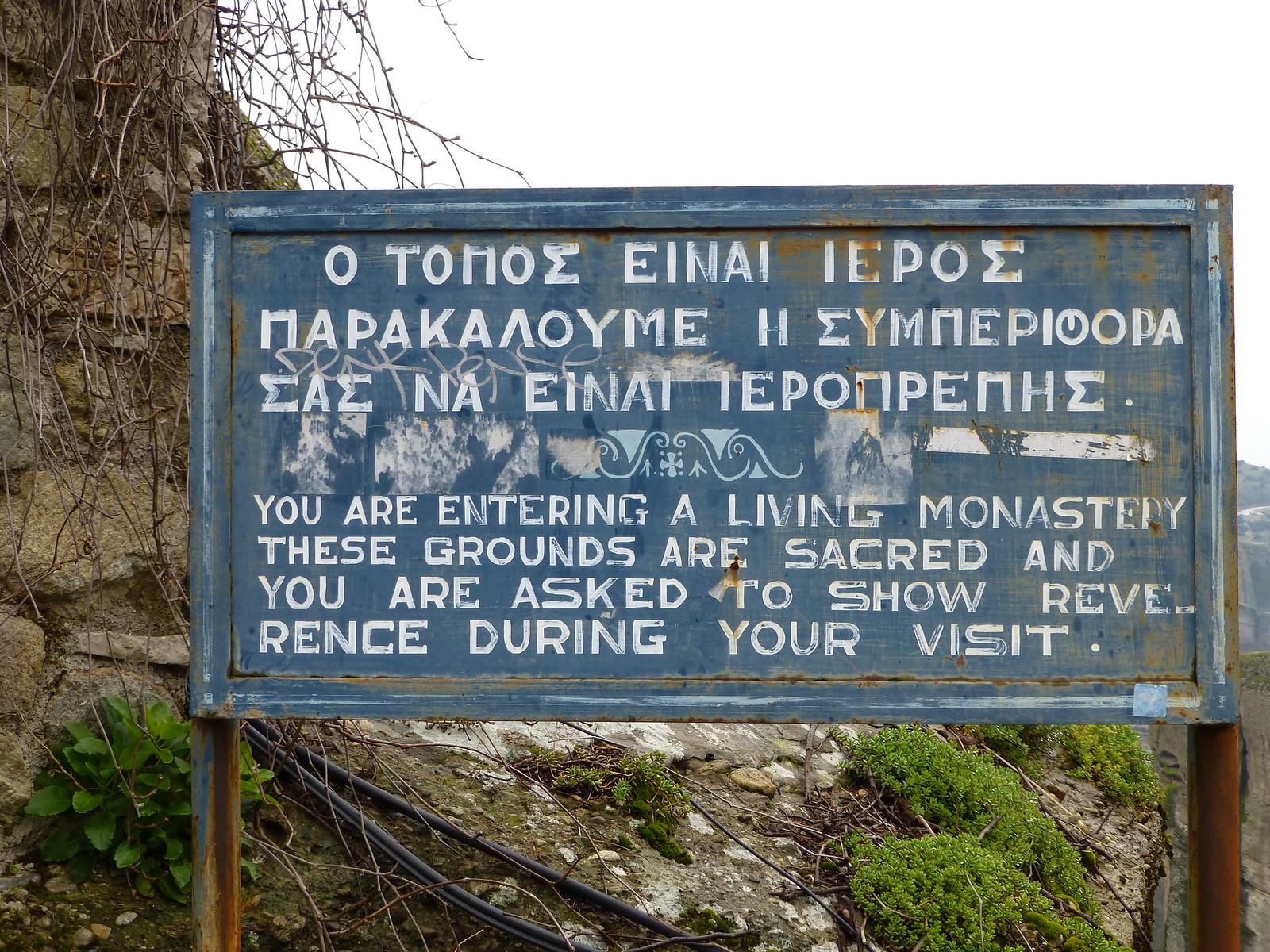In the image, a weathered, blue sign stands slightly off-center to the right, held up by two rusted metal poles against a backdrop of rugged, rocky terrain. The top half of the sign features three lines of text in a foreign language, likely Greek, while the bottom portion in white English letters reads: "You are entering a living monastery. These grounds are sacred, and you are asked to show reverence during your visit." The blue sign, marred by rust and age, contrasts with the gray rocks and the brown of the surrounding branches. Green leaves and plants peek out from below the sign, adding splashes of color to the scene. The background is filled with additional rocks, branches on the left, and a white, overcast sky that looms above. The image appears to have been taken at the foot of a hillside, capturing the rustic and tranquil atmosphere just outside the monastery grounds.